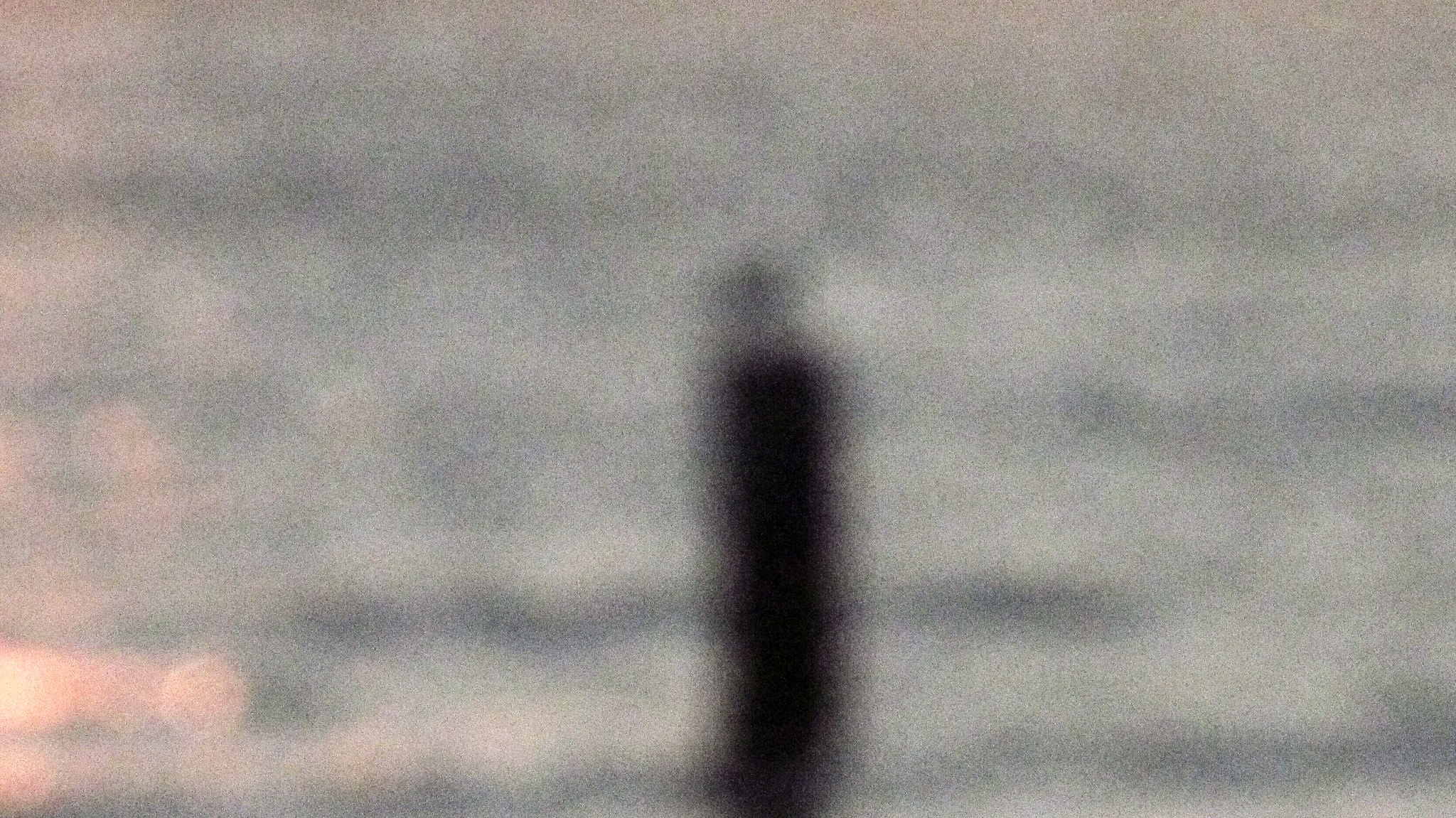In this very blurry and fuzzy photograph, a grayish, square-like figure resembling either a person or a post stands prominently in the center, clad or shaded in black. This figure has a round head that attaches to a squarish body through a thin neck. The image depicts an outdoor setting with what appears to be a waterway in the background. The photograph is horizontally longer than it is vertically, with a mottled and flecked backdrop of gray and off-white hues. To the right of the figure, the background displays gray tones with some black lines, while the left side features a lighter pink shade interspersed with lines of black. In the bottom left-hand corner, a subtle geometric shape emits hues of pink, orange, and red, adding a touch of sunset color to an otherwise muted and indistinct scene. The overall impression is that the photo was taken with a zoomed-in or fuzzed-out focus, making it difficult to discern precise details.